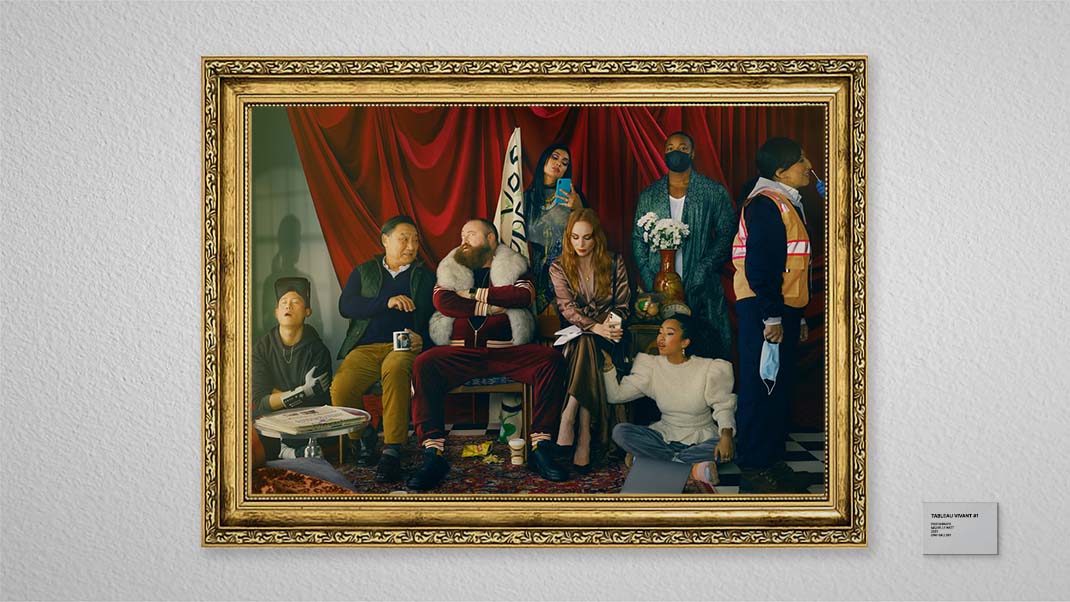In this exquisite painting, prominently displayed in a luxurious gold frame on a pristine white wall, several figures are meticulously depicted, each bringing a unique element to the ensemble. The scene is populated by both standing and seated individuals, with a distinct air of intrigue as some don masks. Among these characters are three females, each adorned in attire that harkens to different stylistic eras. One female, seated on the floor, wears a casual white shirt paired with blue jeans, contrasting starkly against the background. Another female, with striking red hair, is elegantly poised in a brown dress, her demeanor suggesting a classical grace. A figure of notable presence is a robust man clad in a track suit and accented by a white fuzzy vest, adding a contemporary touch to the tableau. The entire scene is set against the dramatic backdrop of a large red curtain, which adds depth and a sense of theatricality to the overall composition.